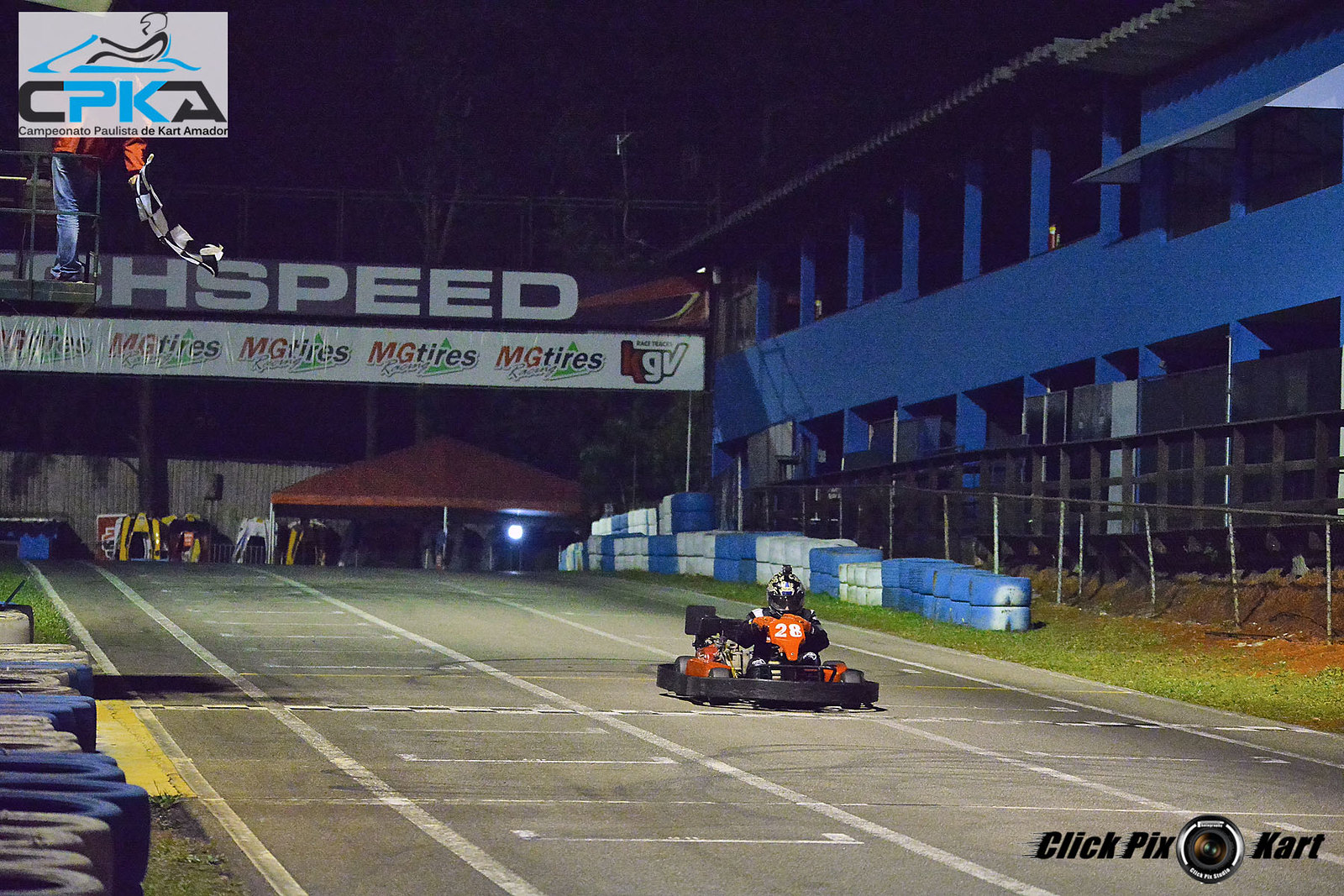The photograph, taken at night, depicts a go-kart racetrack illuminated by artificial light against a backdrop of black sky. Dominating the image is a gray asphalt raceway featuring white stripes, lined with tire barricades painted in various colors, predominantly blue and white. Central to the scene is an orange-colored, open go-kart with red elements, distinguished by the white number 28 on its front. Positioned on the raceway, which appears to slope downward near the starting line, the go-kart has low rails around its perimeter. The driver is suited up in a flame-retardant racer’s jumpsuit and helmet, which is equipped with a GoPro for capturing the high-speed action. At the bottom left and right of the image, tires are arranged on their sides along the track’s edge. The adjacent building in the top right corner, painted blue and topped with a corrugated roof, adds to the setting's ambiance. Toward the top left of the photo, a finish line or checkpoint is marked by white text on a dark background and sponsor logos on a white backdrop. The bottom right corner bears the logo "Click Pics Kart" with a camera lens icon between "Pics" and "Kart."